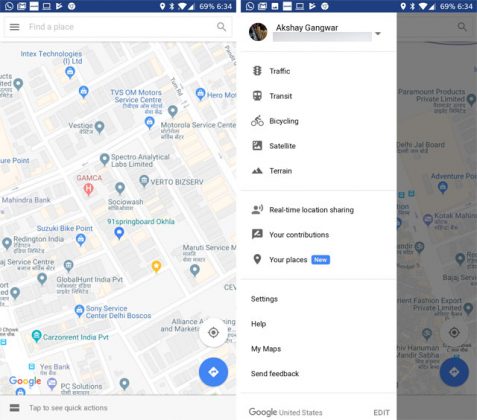The image consists of two side-by-side screenshots from Google-related map features on two cell phones. Both phones have a battery icon in the upper right-hand corner, each indicating a 69% charge. In the first screenshot, a map is displayed with numerous highlighted locations and a yellow bubble with a white star denoting the user's current position. This map showcases various points of interest corresponding to a recent search. The second screenshot reveals a "Your Places" section, where the user has marked specific locations they wish to visit. Above the icons, the user’s name is displayed, providing a personalized touch to the interface. The second screen also includes a series of icons that offer additional information pertinent to the user's searches and saved places.